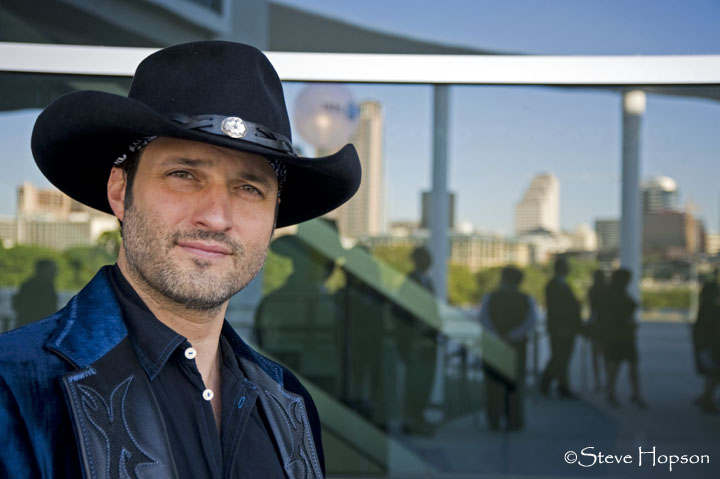The photograph captures a man standing outdoors under blue skies, wearing a black cowboy hat and a matching black leather cowboy jacket paired with a black collared shirt. Sporting a scruffy beard, he strikes a confident pose angled towards the camera, which prominently captures his facial features and attire. In the background, a glass office building reflects the bustling city environment, possibly a place like Dallas, with people milling around and green trees punctuating the urban scenery. The daytime light casts a natural vibrancy over the scene, which includes a blend of colors such as black, white, green, tan, and blue. The photograph is subtly signed "Steve Hobson" in the lower right corner, hinting at the photographer's identity.